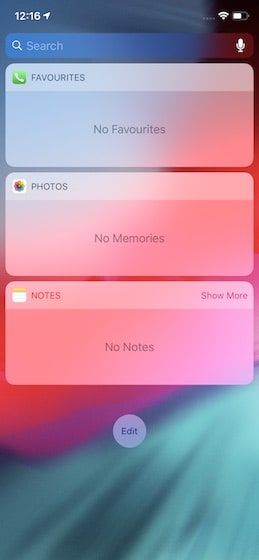Here is a more detailed and cleaned-up caption:

---

A vibrant and colorful screenshot from a cell phone screen captures an array of stunning hues in the background. Predominantly, the center features a mix of reddish-pink tones and a rich fuchsia, interspersed with shades of purple. Teal and gray emerge subtly, particularly toward the top, transitioning into a bluish-gray tint. This diverse palette creates a visually appealing backdrop.

At the top of the screen, white text displays the time as 12:16, accompanied by a partially filled battery icon on the right, estimated at about 75% capacity. Next to it, the Wi-Fi connectivity icon confirms the device is online. Below, a search bar stretches across the screen, ending with a microphone symbol indicating voice search functionality.

In the top corner of the screen sits a green phone icon within a box labeled "Favorites," which currently states "No favorites." An icon representing the photos app—a colorful flower—indicates "No memories" beneath it. Additionally, a notes section appears, showcasing a small calendar with the option to "Show More," but it indicates there are "No notes" at present. At the very bottom, a gray "Edit" button allows for modifications to the displayed widgets.

---

This caption provides a comprehensive and vivid description of the cell phone screen, incorporating all subtle details and ensuring clarity.